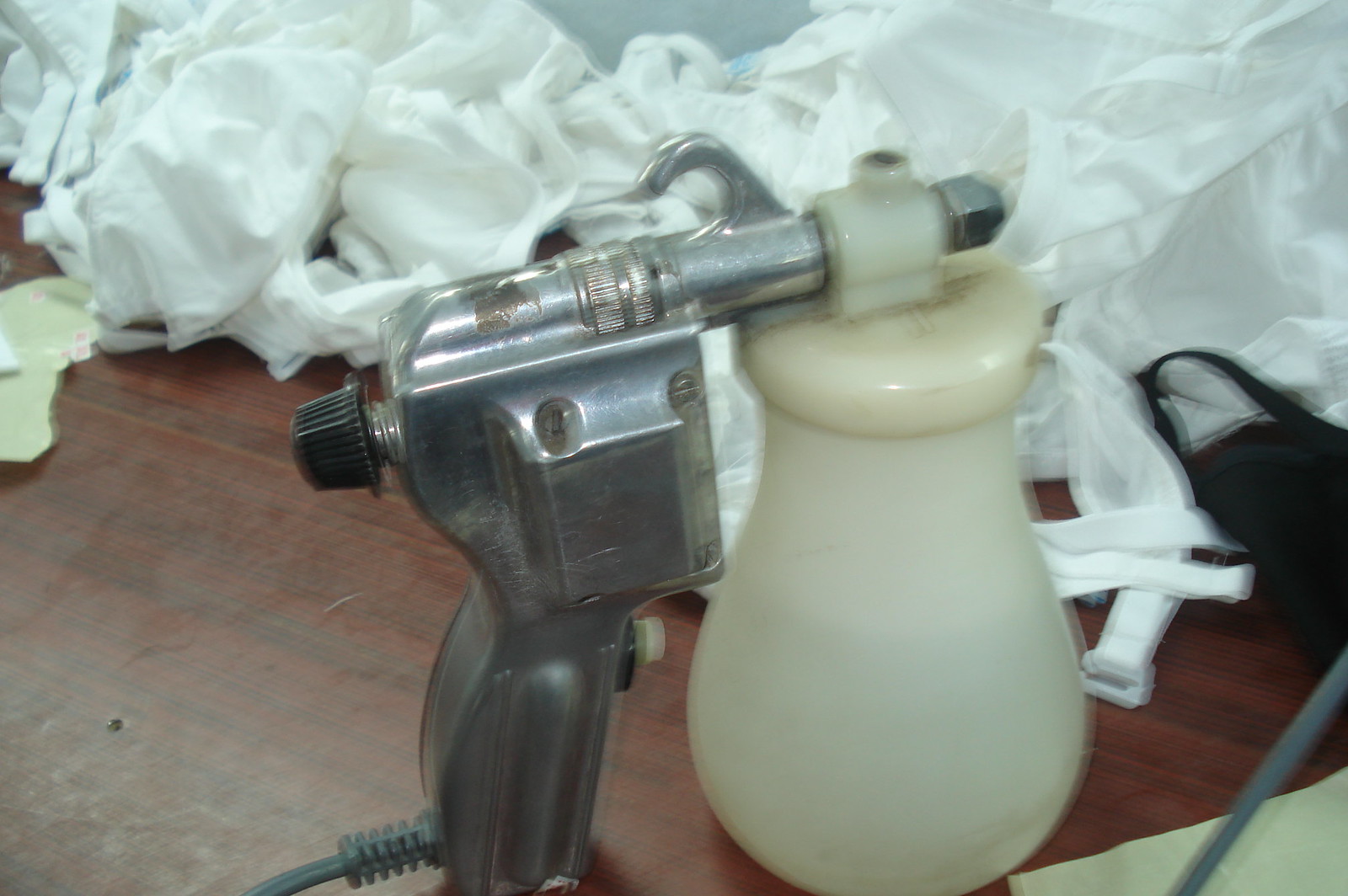In the photograph, we see an old, metallic spray paint gun resting on a floor that appears to be rosewood, characterized by auburn maroon hues and black streaks. The spray gun is silver in color with an angular housing wider than the handle, which boasts a gun-like trigger. Attached to the barrel towards its end is a dark, obtuse plastic container, serving as a paint reservoir, hanging via a plastic loop. The gun is equipped with a ridged black knob at the back and a hex nut at the front end, with a gray cord emerging from behind.

Surrounding the spray paint gun are several white crumpled sheets or cloth, possibly protective outfits, distinguished by their straps and fastening buckles. To the right of the spray gun, a piece of paper lies on the floor. Additionally, a black mask is also partially draped over the wood and atop one of the white crumpled sheets.